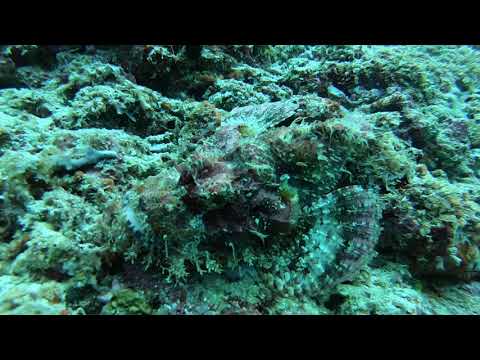This full-color, horizontally rectangular photograph, bordered by black bands at the top and bottom, captures an underwater scene on the ocean floor. It showcases a rich array of coral formations, predominantly in shades of greens and purples, creating a textured and vibrant backdrop. At first glance, the photograph may seem to solely feature the intricate coral, but a closer inspection reveals a camouflaged puffer fish, subtly blending into its surroundings. The fish, difficult to distinguish, can be identified by its purplish hue and a clearly visible fin towards the right side of the image's center. The scene, teeming with marine life and natural complexity, exemplifies the realism and detailed beauty characteristic of underwater photography.